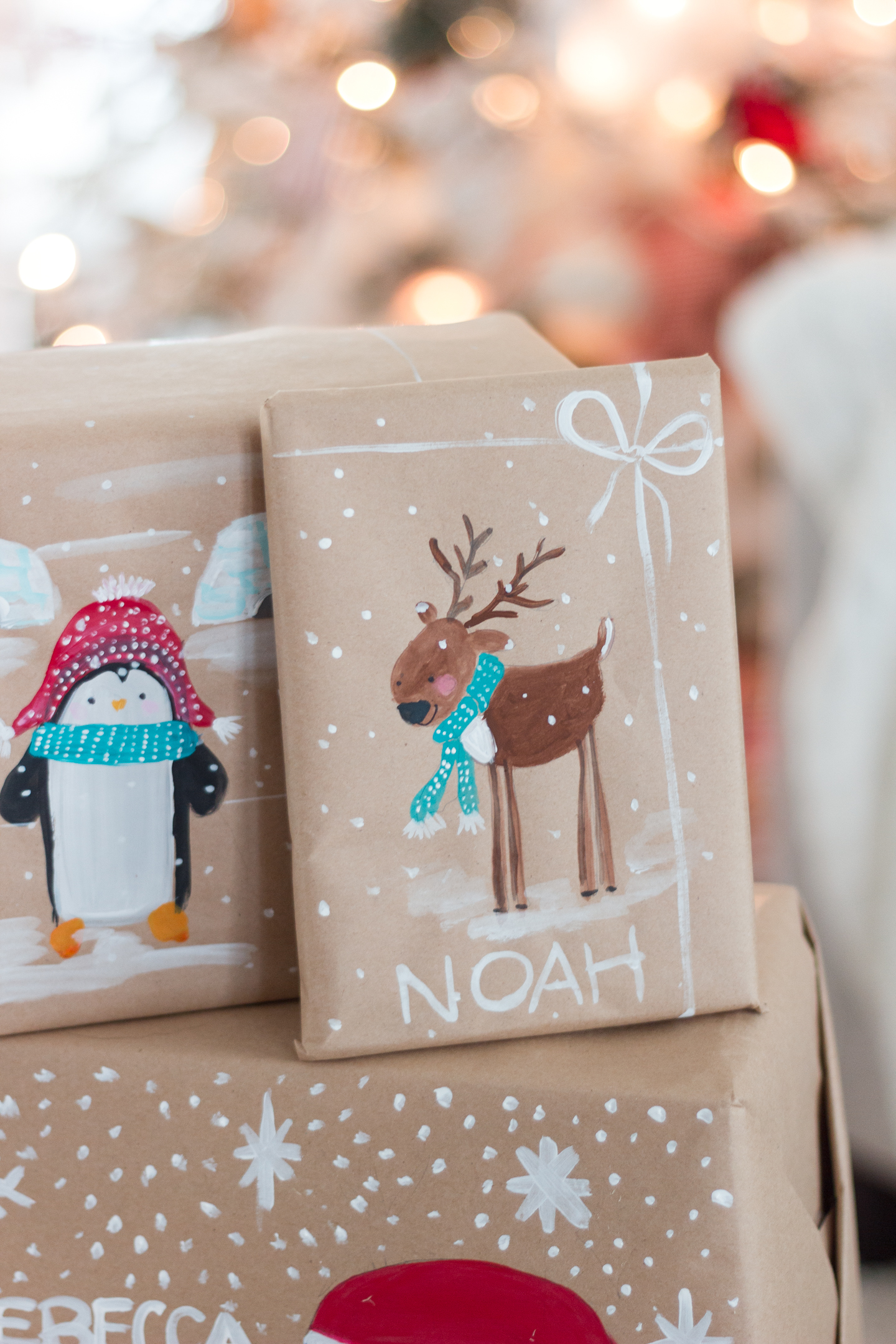The photograph captures a festive scene of Christmas presents arranged on a table. The focal point is on two smaller packages stacked atop a larger one, all wrapped in light brown paper adorned with white specks resembling snow. The topmost gift, seemingly the size of a book (around 9.5 x 11 inches), features a cheerful cartoon reindeer with a brown body, black facial features, rosy cheeks, and two antlers. The reindeer is looking to the left and wearing a light blue scarf with white dots. This present is labeled "Noah" in white letters. Behind it, a second, square package displays a cartoon penguin with a white belly, black flippers, and orange legs. The penguin also sports a light blue scarf with white dots and a red-and-white knitted winter hat with tassels. This package complements the reindeer-themed wrapping. Both smaller gifts rest on a larger parcel, partially visible, which may also feature festive imagery given hints of a red hat and the name "Rebecca" partially in view. The backdrop is softly blurred, highlighting twinkling orange and white Christmas lights and possibly a decorated tree, enhancing the cozy holiday atmosphere.